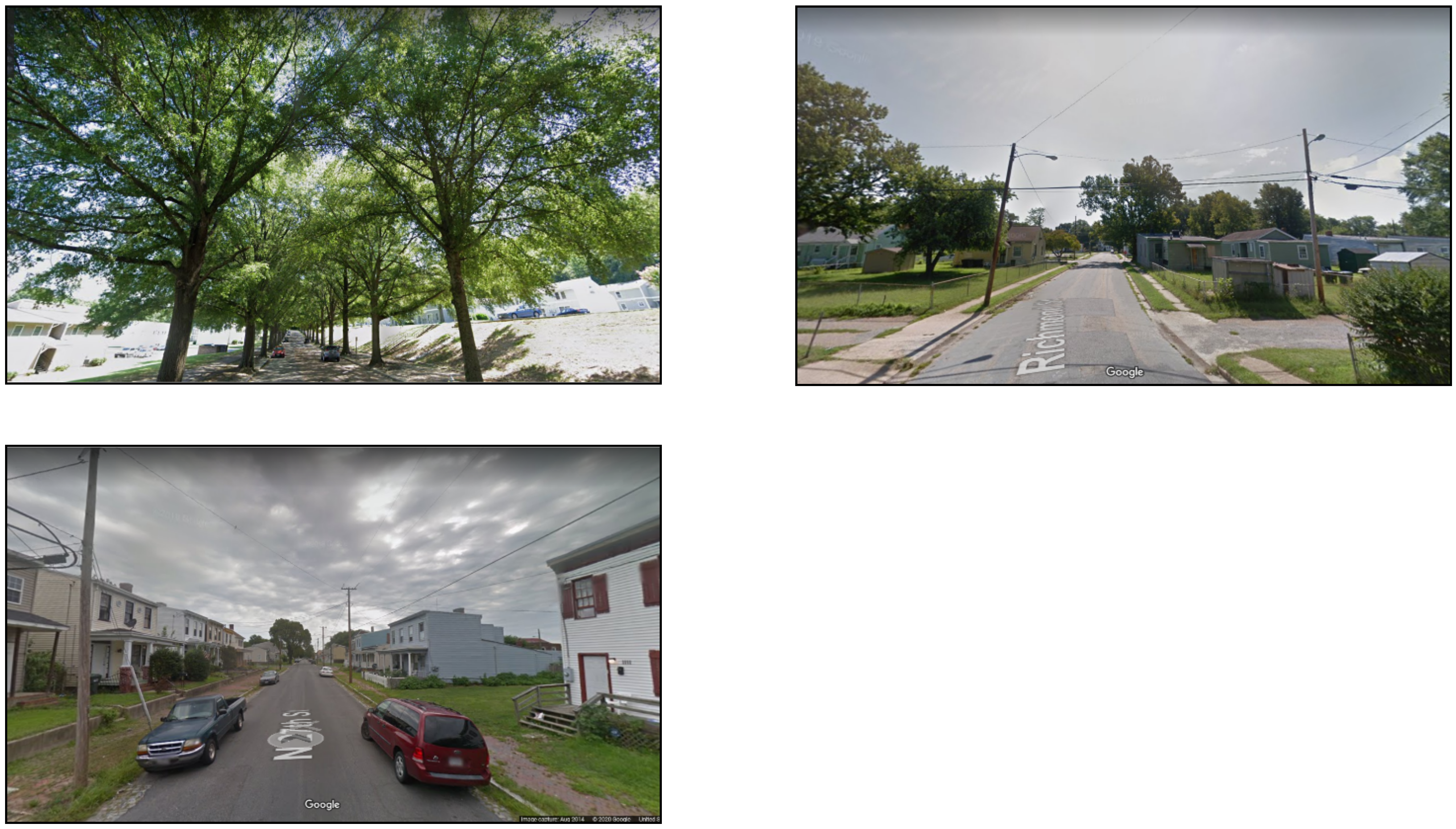This is an image montage of three Google Maps street view photos, arranged on a white piece of paper. The photo in the upper left corner showcases a tree-lined street with deciduous trees forming an arch over the road, casting deep shadows. Cars are parked sporadically along the sides, and a few houses with varying architectural styles are visible in the background. Bright white patches dominate the area under the trees, likely due to overexposure. The top right photo, labeled "Richmond Street" at the bottom, captures a lower-income neighborhood. This area features a mix of trailer homes, overgrown sidewalks, wired gates, and scattered bushes. Above-ground power lines crisscross overhead, adding to the scene's neglected feel. The final photo, located in the bottom left corner and labeled "North 27th Street," presents another modest neighborhood. This scene includes two-story houses closely packed together, separated by narrow grassy front yards. Vehicles like an older model blue car and a burgundy SUV are parked along the street, and telephone poles line the thoroughfare. Overall, the images offer a glimpse into different urban and suburban environments, each with its unique texture and detail.